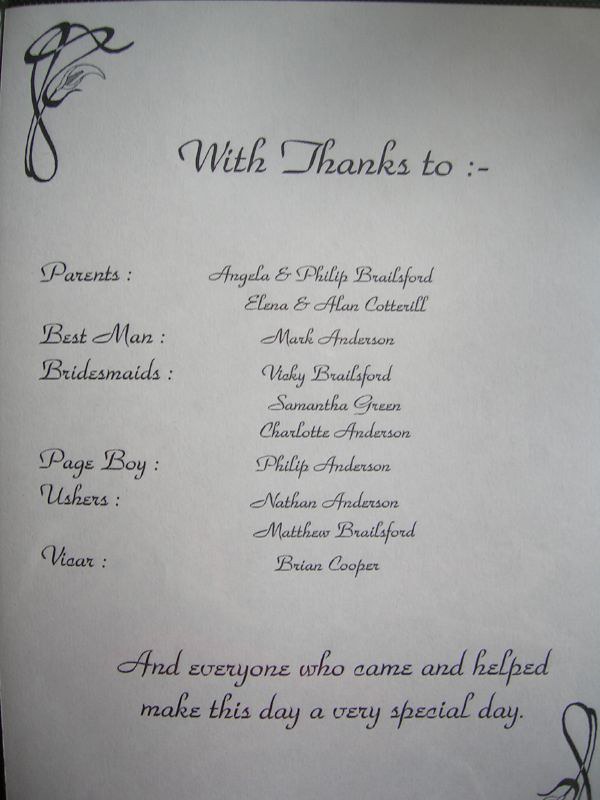The image features a thank-you note printed on a white sheet of paper in a cursive but printed font. The black text expresses gratitude to various individuals who contributed to a wedding. It reads: "With thanks to parents Angela and Philip Brailsford, Elena and Alan Cotterhill, best man Mark Anderson, bridesmaids Vicky Brailsford, Samantha Green, Charlotte Anderson, page boy Philip Anderson, ushers Nathan Anderson, Matthew Brailsford, vicar Brian Cooper, and everyone who came and helped make this day a special day." In the top left corner and the bottom right corner, identical decorative designs resembling an ampersand ending in a small leaf are printed in the same color ink as the text.